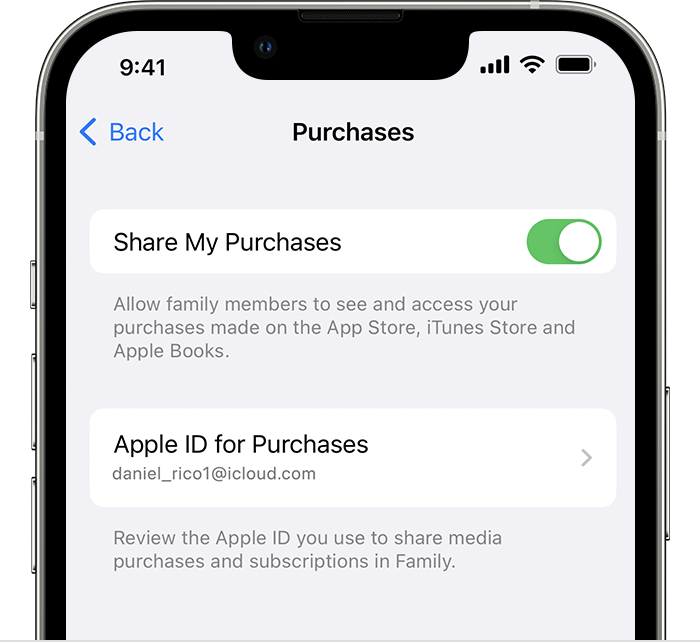A screenshot displays various settings related to sharing purchases on an Apple device. At the top left corner, the time is shown as 9:41. Below that, a blue "Back" button with an arrow pointing to the left is visible. The main focus of the screenshot is on a setting titled "Share My Purchases," which is activated as indicated by the green-shaded toggle bar with a white circle positioned to the far right.

The description under "Share My Purchases" reads, "Allow family members to see and access your purchases made on the App Store, iTunes Store, and Apple Books." Further down, there is another section labeled "Apple ID for Purchases" with an arrow pointing to the right, leading to more detailed settings. The Apple ID associated with this account is daniel_rico1@icloud.com. A note advises the user to "Review the Apple ID you use to share media purchases and subscriptions in Family Sharing."